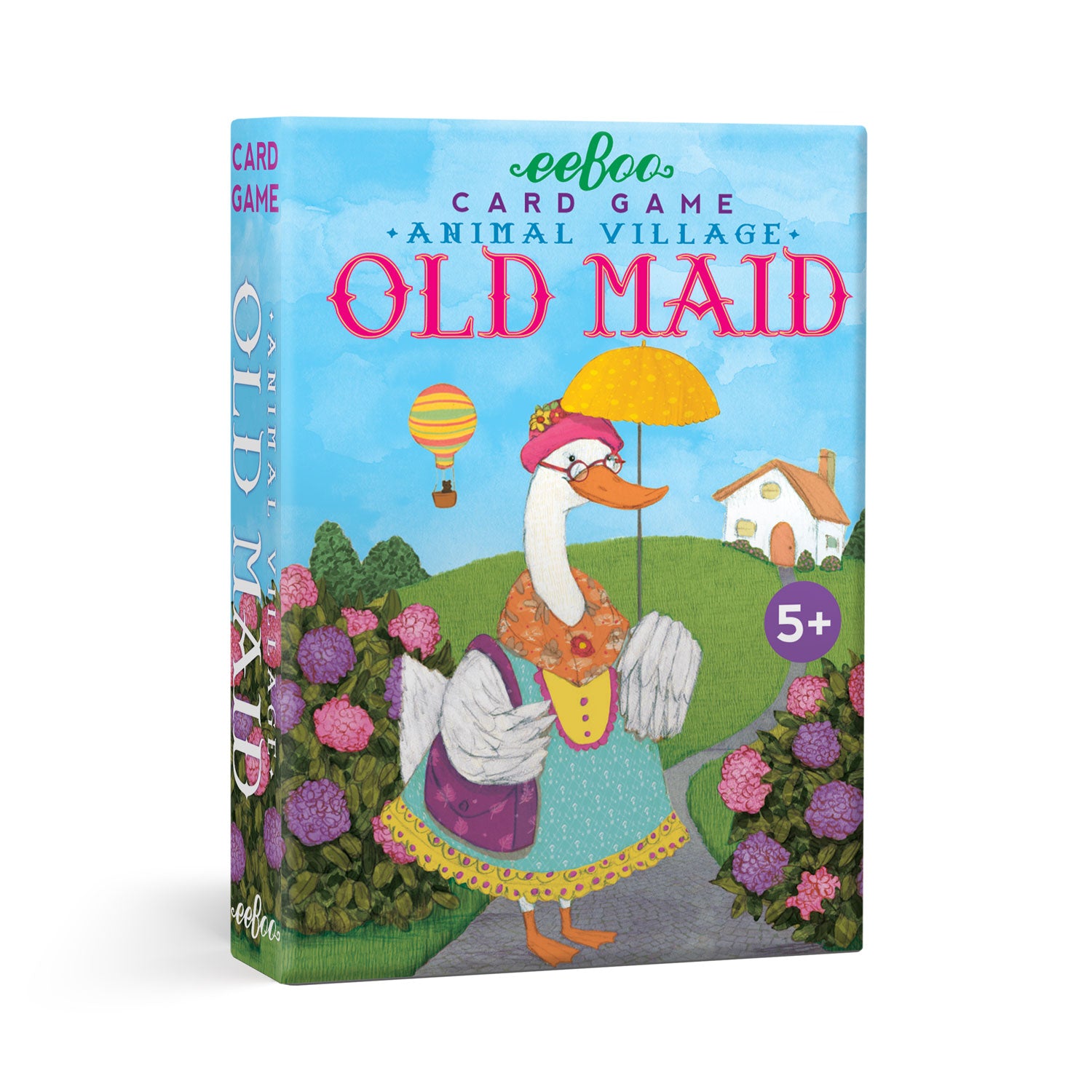The image is a detailed color illustration on the portrait-oriented package cover for the classic card game "Old Maid." The brand name "EEBOO" is prominently displayed at the top in a green script font. Below it, in purple text, are the words "Card Game," followed by "Animal Village" in blue. The largest text on the cover, "Old Maid," is written in pink.

The illustration on the front features an anthropomorphic white duck adorned in an aqua-colored dress, a floral orange scarf, and a pink hat with flowers. The duck has an orange bill and feet and holds a yellow polka-dotted umbrella. It also carries a purple-patterned purse on its shoulder. The duck stands on a gray path that meanders through green grass and leads to a small white cottage with an orange roof and door on the right side of the image. The scene is flanked by blooming hydrangea bushes in pink and purple hues. Overhead, the sky displays a hot air balloon in orange, yellow, and green.

On the right front side of the package, there's a round purple sticker indicating "5+" in white text, denoting the recommended age for players. The background of the upper half of the package is blue, transitioning to green in the lower half, enhancing the vibrant, whimsical setting of the product's artwork.